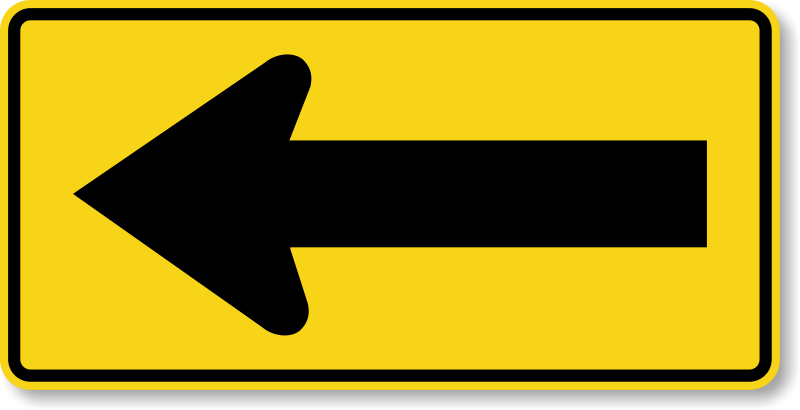The image features a prominently yellow, rounded rectangular road sign that occupies the entire frame. The sign includes a black outline framing its edges, complemented by a shadow cast towards the bottom and right sides, adding a sense of depth. Dominating the center of the sign is a large, black left-pointing arrow, stretching from the right side to the left, making it clear and unmistakable. The overall design, with its bold colors and shapes, gives it the appearance of a clean, vector-based icon or clipart image often used in graphic design, evoking the kind of directional signage typically seen in the United States.